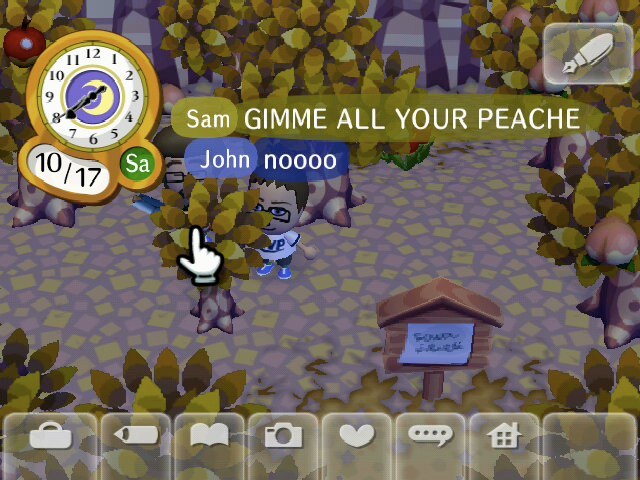The screenshot depicts a scene from a computer game resembling Animal Crossing, set in a whimsical forest environment. Dominating the upper left corner is a clock displaying the date "17 SA" and the time "7:40." Opposite, in the upper right corner, is a transparent square bearing a pen icon. The lower half of the image is lined with semi-transparent icons featuring various symbols including a shopping bag, a pen, a book, a camera, a heart, a speech bubble, a house, and a blank square.

Central to the scene are animated characters among cartoonish trees with yellow and olive-colored leaves. One tree, named Sam, has a speech bubble requesting peaches ("Sam: Give me all your peach"), to which another character, John, responds emphatically with "Nooooo!" This interaction is highlighted by an in-game cursor shaped like a hand, pointing towards the speaking tree. Additionally, there is an unreadable signpost placed in front of the characters, enhancing the game's immersive environment.